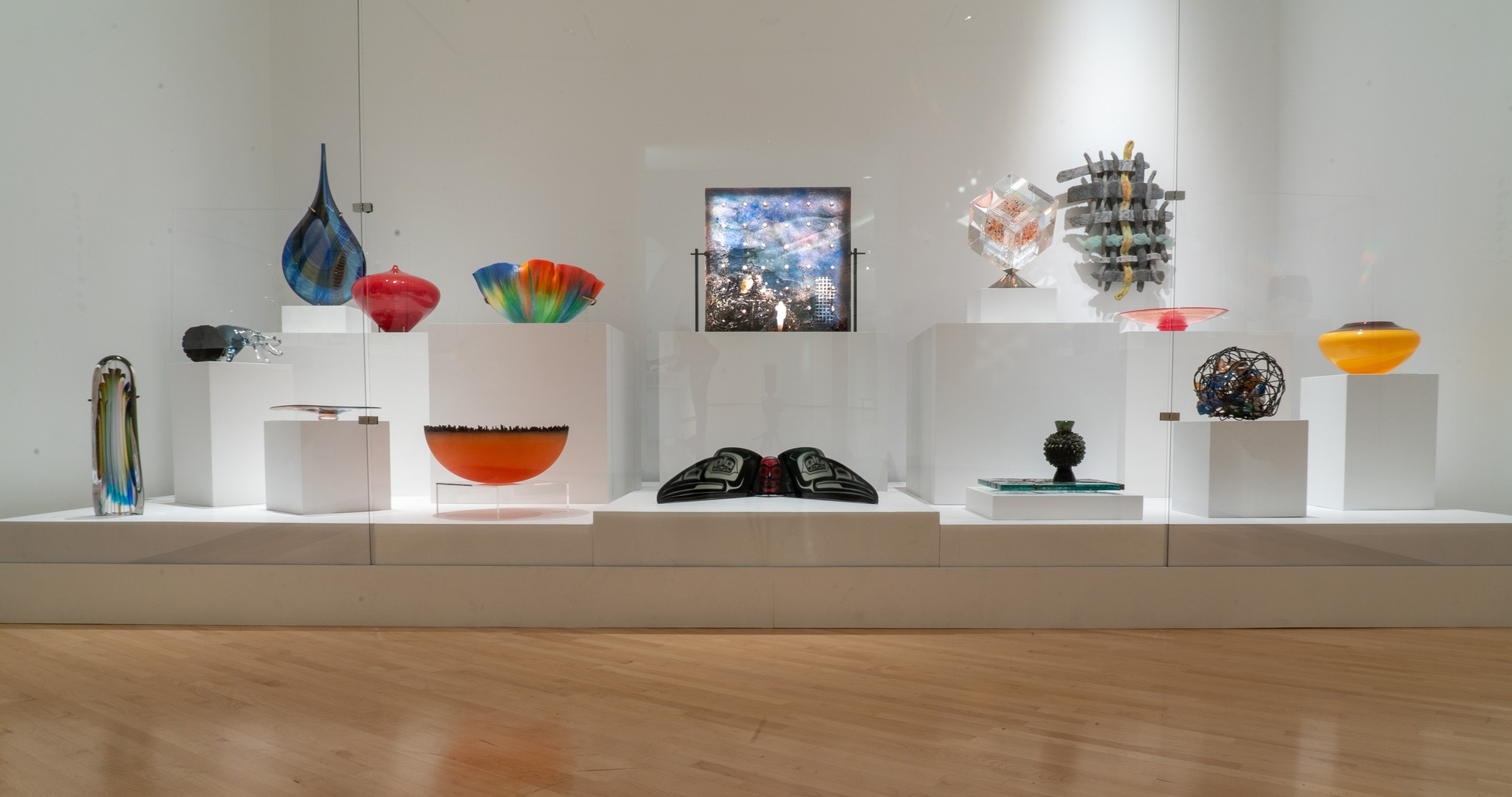The image captures a polished, light-colored hardwood floor with a glossy finish, reflecting its well-maintained condition. In the background, there is a small, foot-high ledge acting as a platform. On this platform stand several tall, white rectangular pedestals, serving as display stands for various abstract art pieces. Among these art objects, on the left, you can observe a blue vase, a red vase, and what appears to be a rainbow-colored container. Further to the right, there is an orange bowl accompanied by another circular design, and a lit-up screen or panel positioned in the middle. The pristine white walls of the room ensure that the colorful artwork stands out prominently. Although a white and blue item, possibly a water bottle, is visible near the left edge, it remains unclear in purpose. The image lacks any human presence or text, focusing solely on the art display within this bright, modern exhibit space.